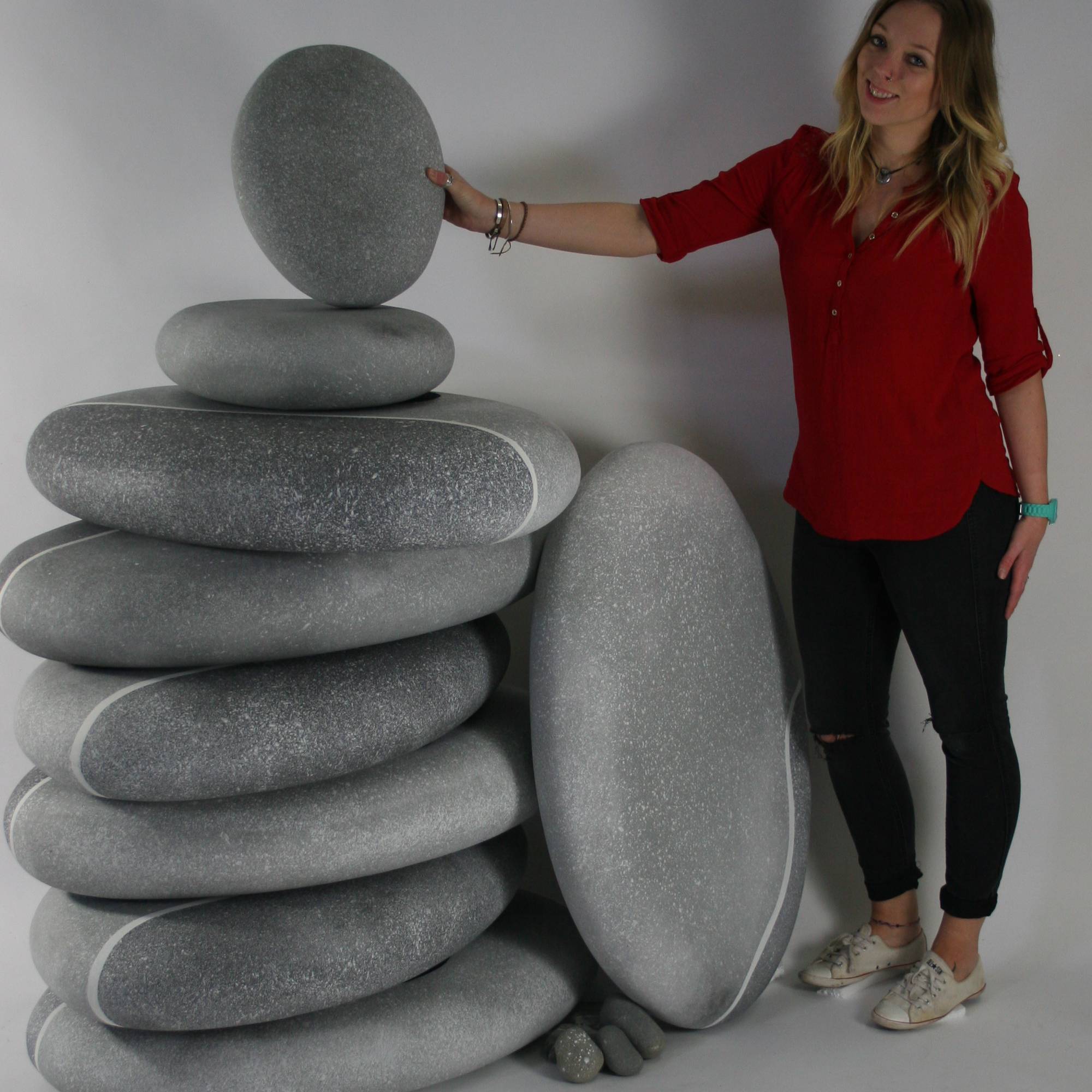The color photograph captures a smiling, blonde-haired woman who appears to be about 30 years old. Dressed in a red blouse, black pants, and white converse-style shoes without socks, she accessorizes with a turquoise smart watch and several bracelets on her arm. Her wavy hair frames her face as she stands next to an intriguing art installation, composed of enormous, smooth, gray river pebbles with occasional white stripes. The stack of pebbles, likely made from lightweight materials such as fiberglass or styrofoam, reaches up to her chest and includes about eight to ten stones. She is holding one of these large 'pebbles', effortlessly suggesting it's light despite its large size. Another prominent pebble stands on end near her waist. The scene combines the grace of artistic illusion with the natural appearance of river stones, all brought to life by her engaging presence.